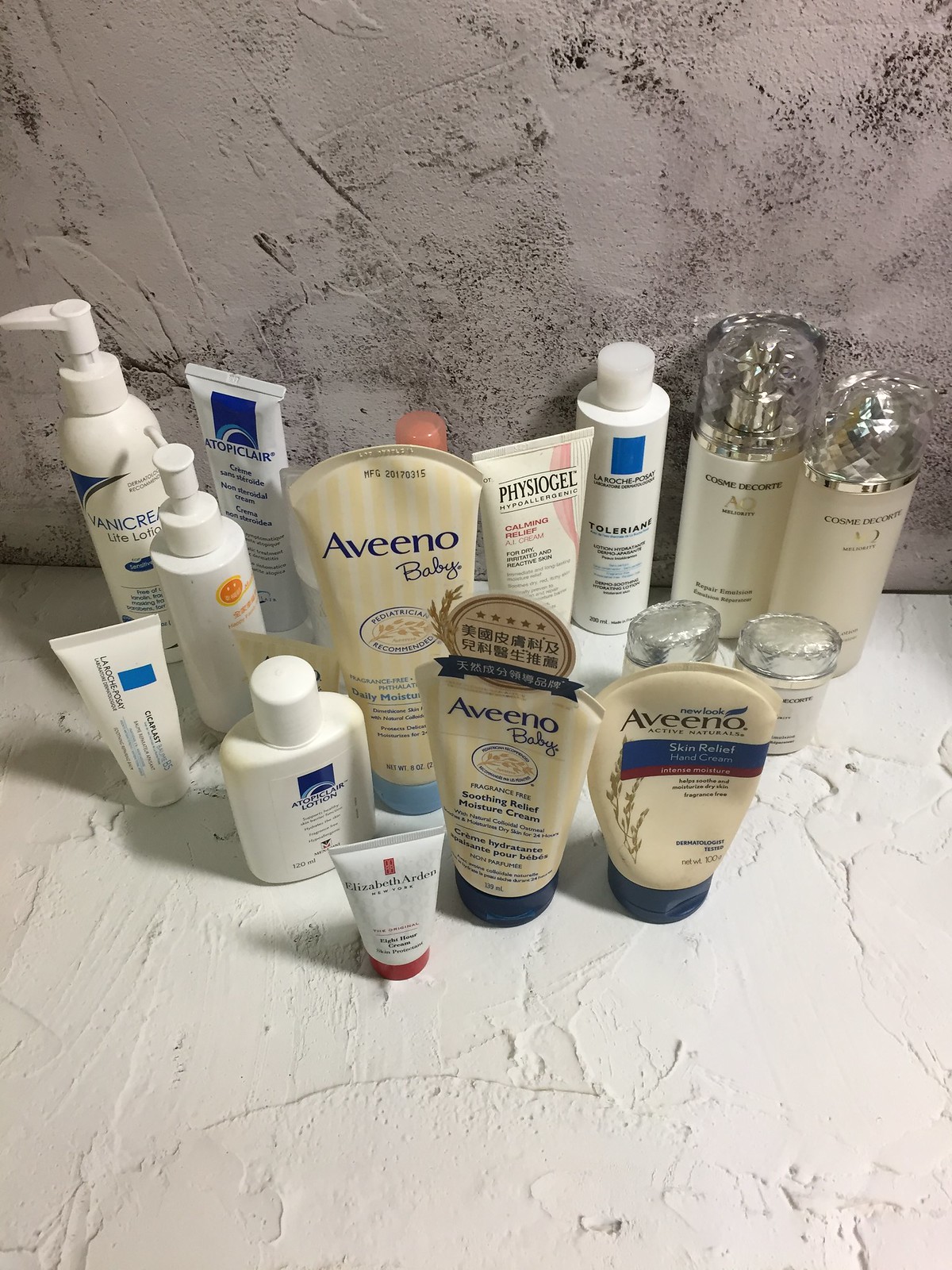The image depicts an artfully arranged collection of beauty products set against a white, textured surface. Behind the display is a light gray wall adorned with black speckles, adding a subtle backdrop to the scene. Central to the arrangement are three distinct products from the Aveeno Baby line, identifiable by their packaging featuring blue text on a pale yellow background. Prominently positioned in the forefront is a tube standing on its cap, bearing the iconic red and white design of Elizabeth Arden. Surrounding these key items are various other bottles of lotion and beauty products, creating a visually appealing display that highlights both brand recognition and the diversity of skincare offerings.